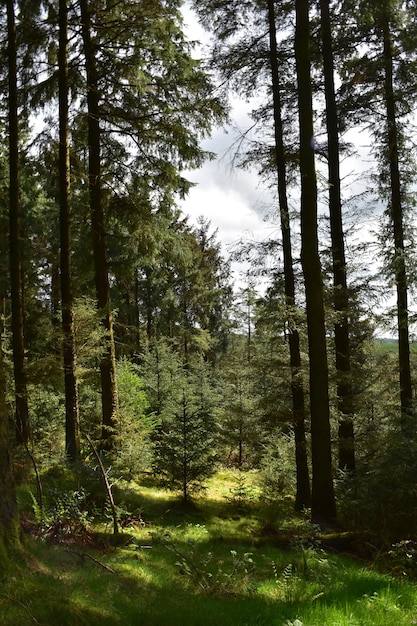This photograph captures a lush forest scene dominated by tall, slender trees with dark brown trunks that stretch upwards towards the sky. Their feathery leaves and green vegetation spread out from their tops. The ground is a vibrant green, covered with grass and small flowering plants, mostly bathed in shade. In the center, younger and smaller trees add variety to the landscape with their bushier appearance. On the right side of the image, more tall, thin trees rise, contributing to the dense forest atmosphere. The background reveals a sky adorned with fluffy white clouds and sunlight filtering through, casting a gentle glow on parts of the forest floor.